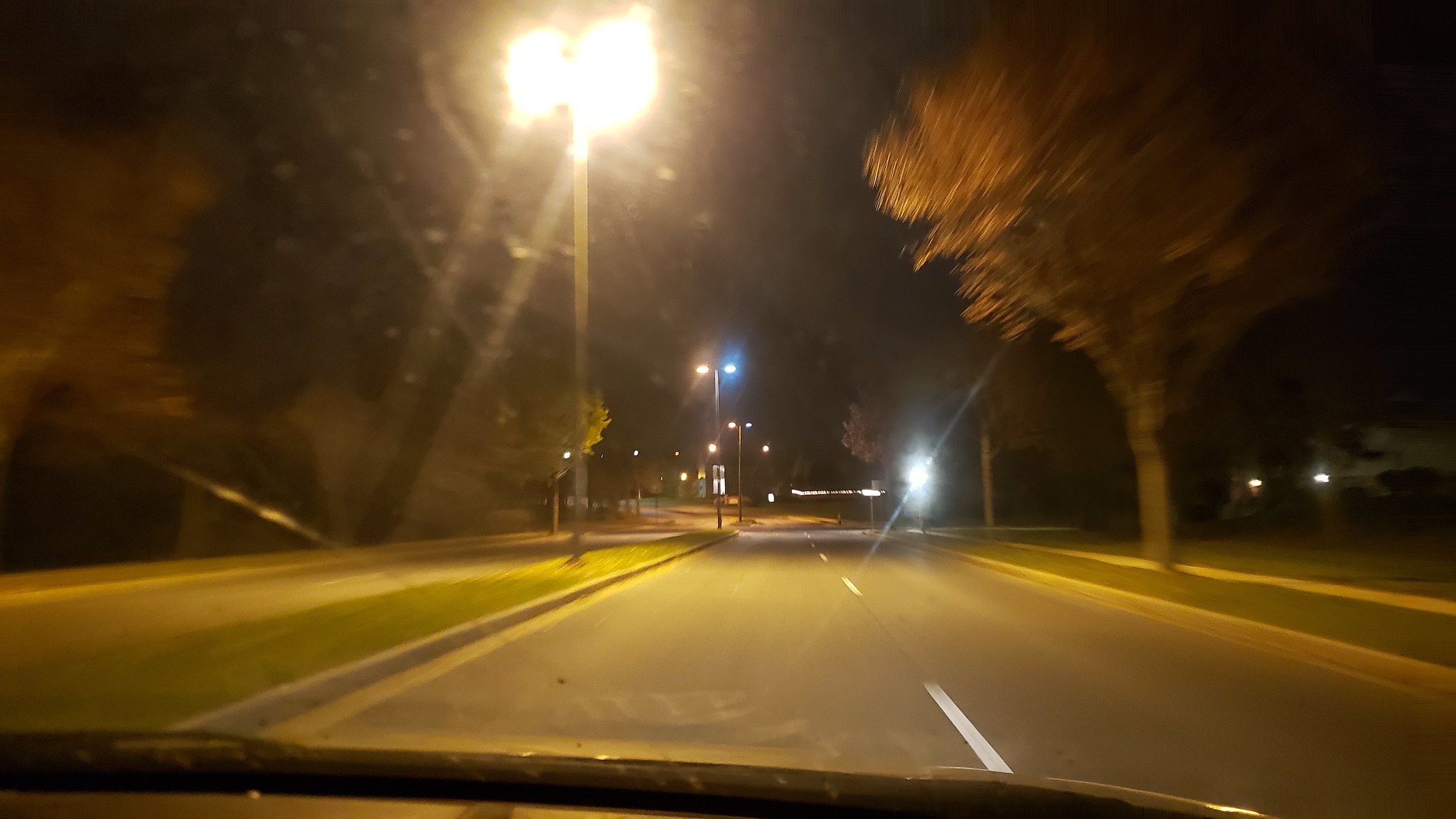A nighttime photograph taken from inside a car shows a dark road divided by a grassy median with two lanes on each side. The road, marked with white lines, stretches ahead under a completely dark sky. On both sides of the road, sidewalks and curbs border grassy areas. To the right, trees display a mix of green and red leaves, illuminated by a series of streetlights lining the road. These streetlights, two per pole, cast a white glow, with some lights appearing bluish due to the blur of motion. Further down the road, there are more trees with similar foliage, and a building with lights can be seen in the distance. The car, positioned in the left-hand lane, reveals a black hood through the windshield. The overall scene is lightly blurred, enhancing the nighttime ambiance.